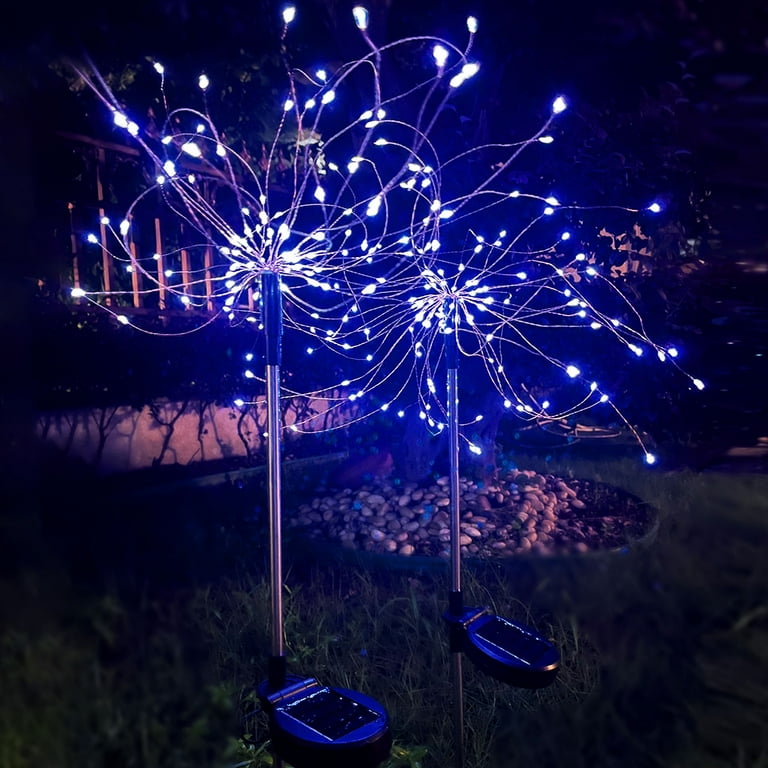This color photograph, taken outdoors at night in a garden setting, displays two solar-powered light fixtures staked into a green, grassy lawn. Each fixture consists of a silver pole topped with multiple stiff, curved wires, which emanate in all directions like an exploding firework. At the end of each wire is a small, brightly lit, bluish or white light resembling delicate flowers or fiber optic strands. Midway up each pole, a noticeable royal blue solar panel captures sunlight during the day to power the lights at night. In the background, a wooden patio fence and a small rock garden, surrounded by a circle of stones, add to the scene's serene ambiance.